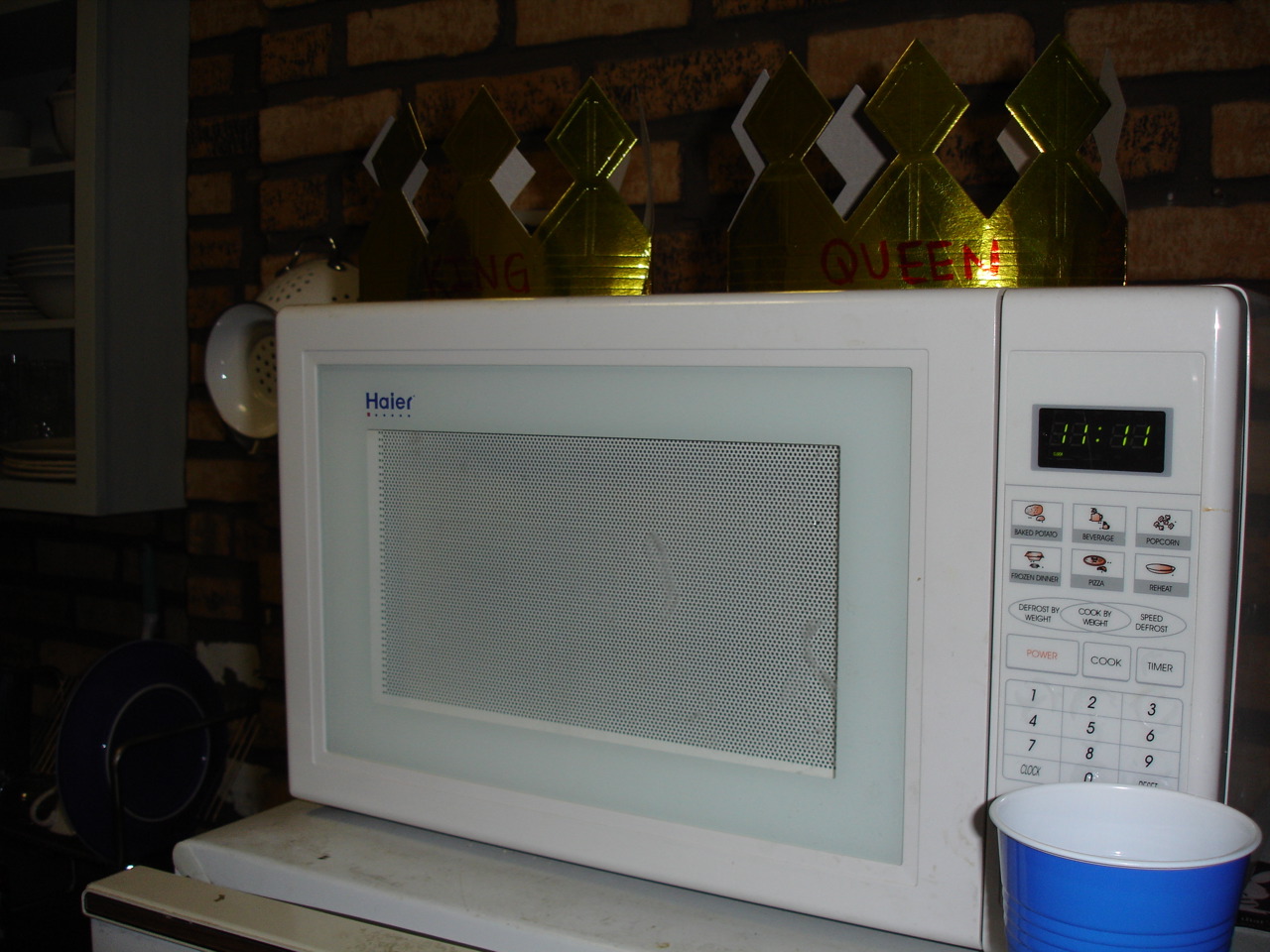This photograph, taken in a dimly lit room, centers on a well-used, white microwave oven branded Haier (H-A-I-E-R). The microwave displays the time 11:11 and is situated on a small refrigerator with a partly open door that features a brown design. The appliance has a transparent door with black dots and an operation pad to the right, where a blue plastic solo cup is placed in front. Two gold crowns, labeled "king" and "queen," rest on top of the microwave. The background reveals a brick wall and some hanging objects, possibly mugs and a teapot or colander, though they are indistinct against the dark surroundings. There is also a shelf on the left holding white plates and bowls. The image is poorly lit, with the light mainly highlighting the microwave and the blue cup, rendering much of the room in shadow.